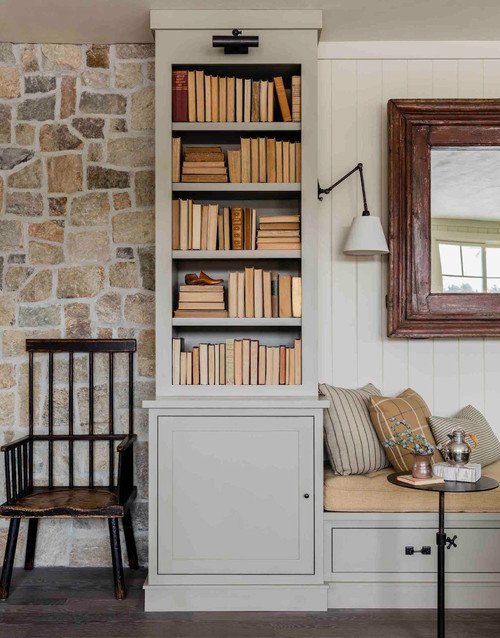The photograph depicts a cozy, indoor seating area within a home, oriented in portrait mode. The left third of the image features a rustic stone wall made of light brown, off-white, light gray stones, bound together with off-white grout. In front of this wall, there's a high-back wooden chair that may have a leather or wood seat resting on a brown floor, giving off a shaker-chair vibe. To the right of the chair, a narrow, ceiling-high bookcase stands, filled with books arranged for decorative purposes—many of the books showcase their pages, in shades of yellow, white, and tan, with notable exceptions of a red and a gold book.

Adjacent to the bookcase is a built-in seating area. The seating includes a white futon adorned with yellow cushions and pillows featuring tan, black, and brown stripes. The area is illuminated by a white and black swing-arm lamp mounted on the wall. Above the futon hangs a large mirror with a brown wooden frame, reflecting windows elsewhere in the room. Below the seating area, white cabinets and drawers with black handles provide additional storage.

In front of this cozy nook, there’s a small black table displaying blue flowers in a gold pot, accompanied by a silver pot set on a white book. A yellow book supports the first pot. The ceiling in this room appears gray, and it holds a black light fixture at the top of the bookcase, highlighting the varied elements of this inviting reading or family room.